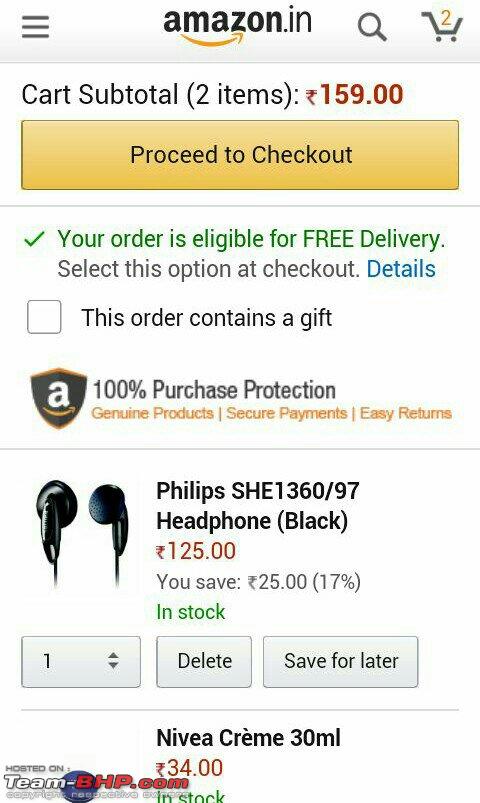The screenshot from Amazon.in features a gray border at the top, displaying the Amazon logo and a magnifying glass icon next to it. Two items are shown in the cart. Just below, on a white background, it states "Cart Subtotal (2 items): ₹159.00." An orange rectangle labeled "Proceed to Checkout" with black text is positioned beneath this. Next, a green checkmark indicates, "Your order is eligible for FREE Delivery," with the instruction, "Select this option at checkout" in black text below it. A clickable link labeled "Details" in blue font is also present. 

To the side, there's an unchecked box next to the option that says, "This order contains a gift." There's a black shield icon with an 'A' in the center, underlined by an orange stripe, followed by the text "100% Purchase Protection - Genuine Products, Secure Payments, Easy Returns."

The product displayed is a pair of black earbuds, specifically identified as "Philips SEH1360/97 Headphone, Black." The price listed is ₹125, reflecting a discount where you save ₹25, which is a 17% reduction from the original price.